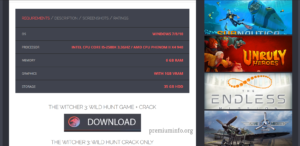The image depicts a user interface of a streaming platform. The website is quite blurry, but several key elements are discernible. A thick, vertical black line runs from the top to the bottom of the screen. To its right, there is a black rectangular box that contains a single column with text, each row displaying a single word. Adjacent to this, in red text, there are five rows of information listed below a header.

At the bottom of the screen, there is a noticeable black download button featuring a logo and the word "Download" prominently displayed in big white letters. The main content being streamed is "The Witcher." 

To the right of this section, another thick vertical black line is present, followed by four distinct boxes, each showcasing an image related to a different movie or video. Another thick black vertical line appears beyond these boxes, sectioning off parts of the interface.